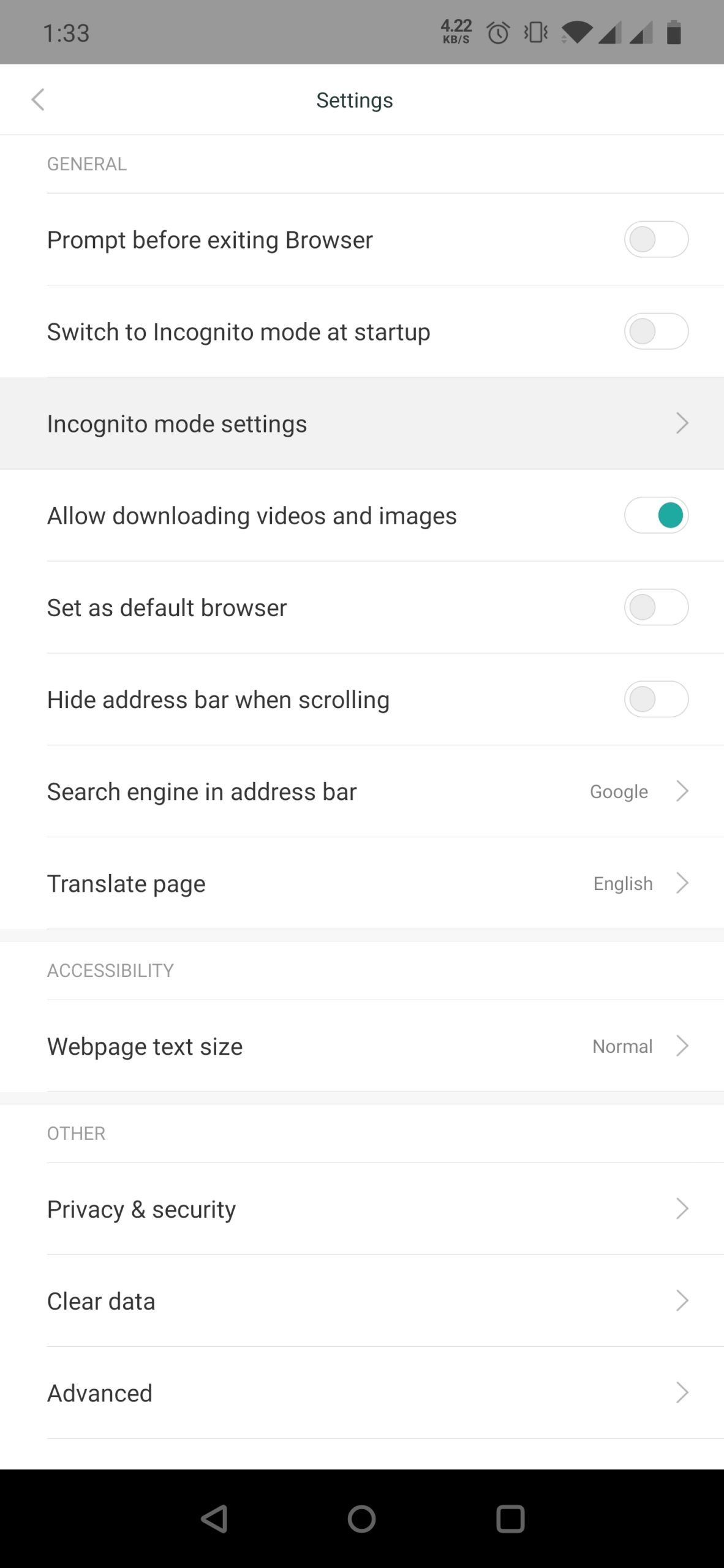Screenshot of a Settings Menu on a Smartphone Browser

At the top of the screen, the time is displayed as 1:33 PM in the top-left corner, while the phone's status indicators, including signal strength, alarm, and vibration status, are shown in the top-right corner.

The main content of the image shows the settings menu of a browser, with a section labeled "General." Within this section, several settings are listed:
- "Prompt before exiting browser"
- "Switch to incognito mode at startup"
- "Incognito mode settings"
- "Allow downloading videos and images" (with the setting toggled on)
- "Set as default browser"
- "Hide address bar when scrolling"
- "Search engine in address bar"
- "Translate page"

Below the "General" tab, there is an "Accessibility" section with the option "Web page text size."

Further down, the menu includes an "Other" section featuring:
- "Privacy and security"
- "Clear data"
- "Advanced settings"

At the very bottom of the screen, there is a black bar containing a back button, a home button, and a square button, presumably for navigating the device's interface.